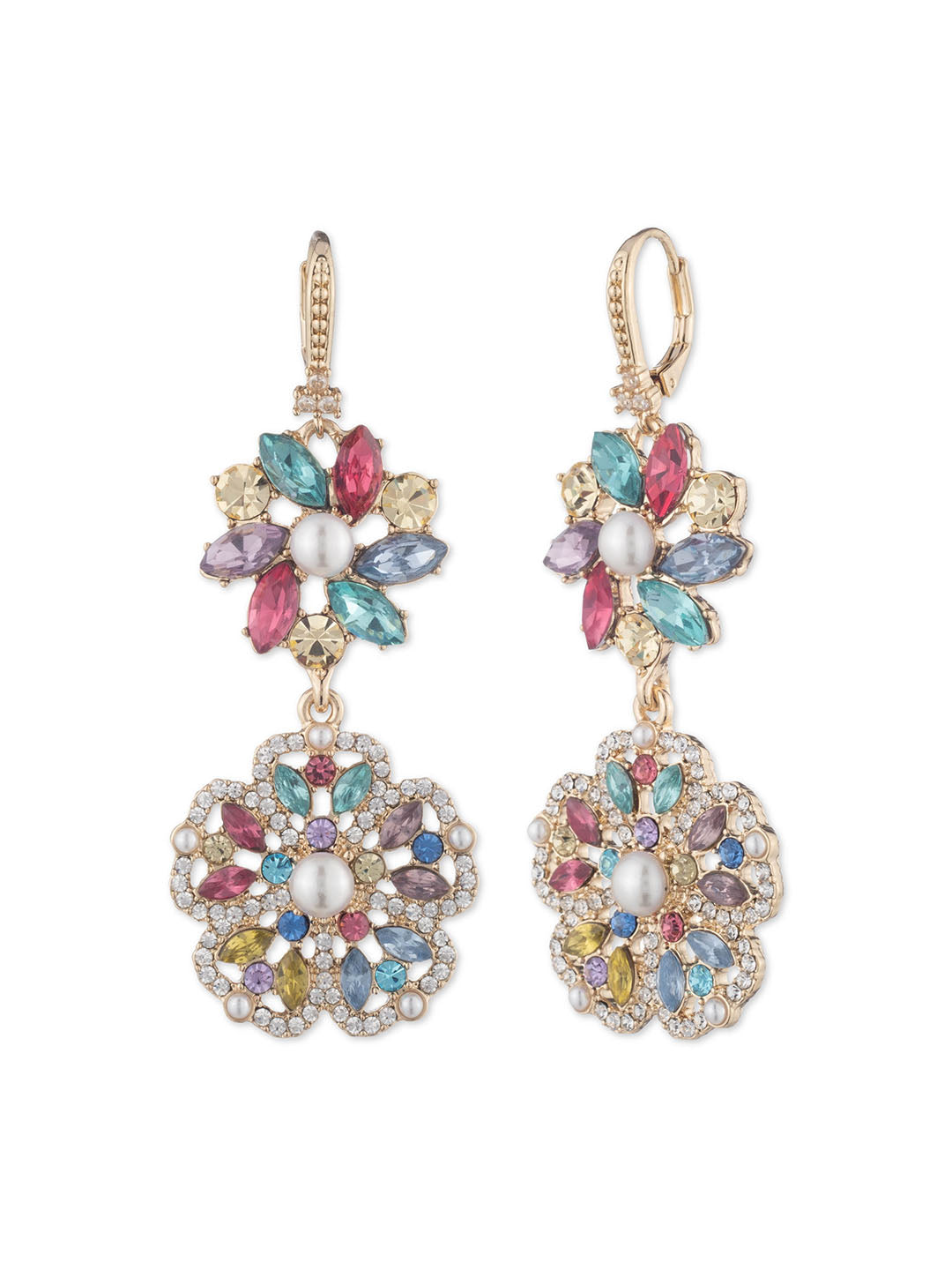This image features a detailed view of a pair of elaborate, vintage-inspired dangling earrings, likely mimicking styles from the 1960s or 1970s. Each earring begins with a gold hoop that serves as the clasp, looping through the ear. Hanging beneath the hoop is an intricately designed flower adorned with an array of multicolored jewels—green, red, purple, and gold pieces interspersed throughout. The center of this floral motif boasts a prominent pearl, complementing the tiny faux diamonds that outline the petals. A second, more ornate flower dangles underneath, outlined in gold with a complex pattern of jewels inside, including green, red, yellow, and brown hues. The middle of this lower flower is also set with a pearl, surrounded by a faux diamond pattern. The earrings are displayed against a plain white background, showing two different perspectives: one earring is depicted face-forward, while the other is slightly angled to reveal its clasp. These two angles highlight the symmetrical placement of the jewels and the intricate craftsmanship of the design.